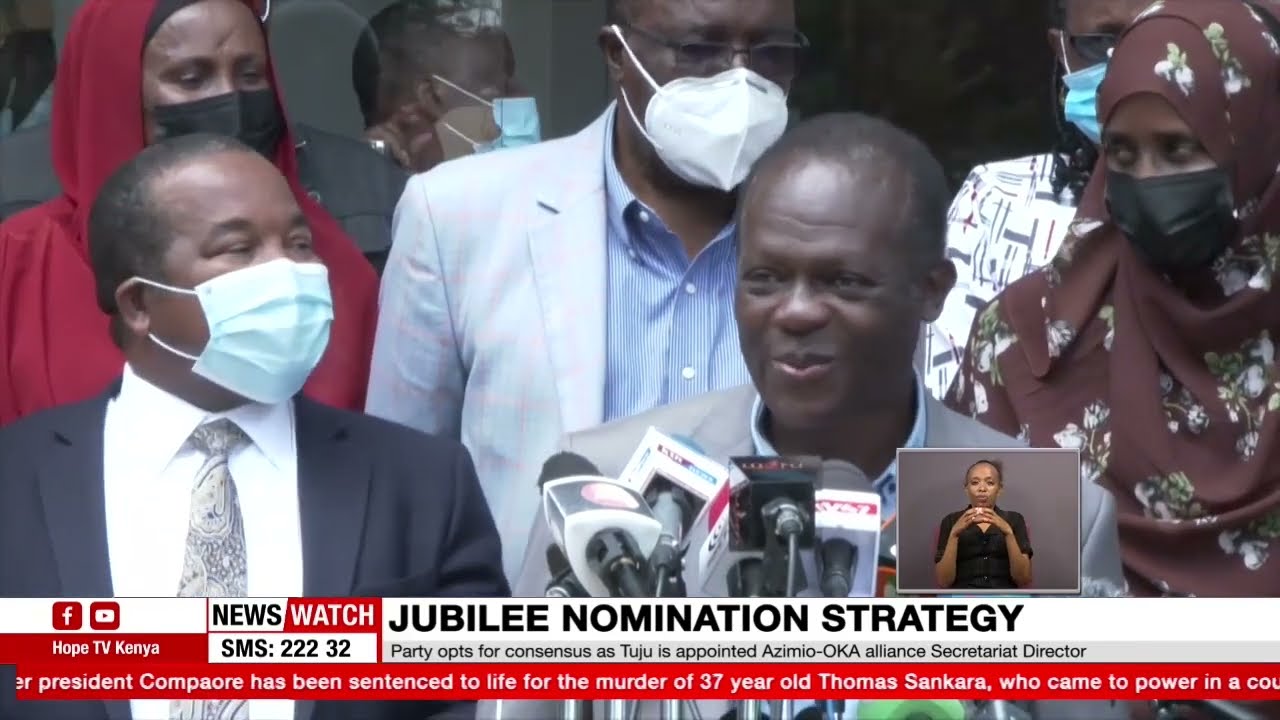The image captures a television newscast from Hope TV Kenya, showcasing a political presentation. At the center of the image, a dark-skinned man dressed in a light gray suit and blue collared shirt stands behind a bundle of microphones. He looks to his right with a subtle smile. In a small pop-up window to the right of him stands a black woman with her hands folded in a praying position, presumably an interpreter for the deaf.

Surrounding the central figure are eight other individuals. Immediately next to him is another dark-skinned man, wearing a dark suit with a white shirt and tie, who looks at the central figure attentively while wearing a mask. Behind these two men, another man can be seen in a light gray or white suit paired with a blue shirt, wearing a mask and glasses. To their left stand two women with head covers and masks; the woman on the left dons a red head covering with matching fabric covering her entire body, while the woman on the right wears a brown head cover and dress adorned with flowers.

In the red and white caption bars below, the primary news items read "News Watch Jubilee Nomination Strategy," with detailed information indicating that the party has opted for consensus as Tuju is appointed Azimio Oka Alliance Secretariat Director. Another red banner informs viewers of a related news story: "President Kampaore has been sentenced to life for the murder of 37-year-old Thomas Sankara who came to power in a coup," although the sentence finishes abruptly. The scene implies the presence of COVID-19 given that most individuals are wearing masks.